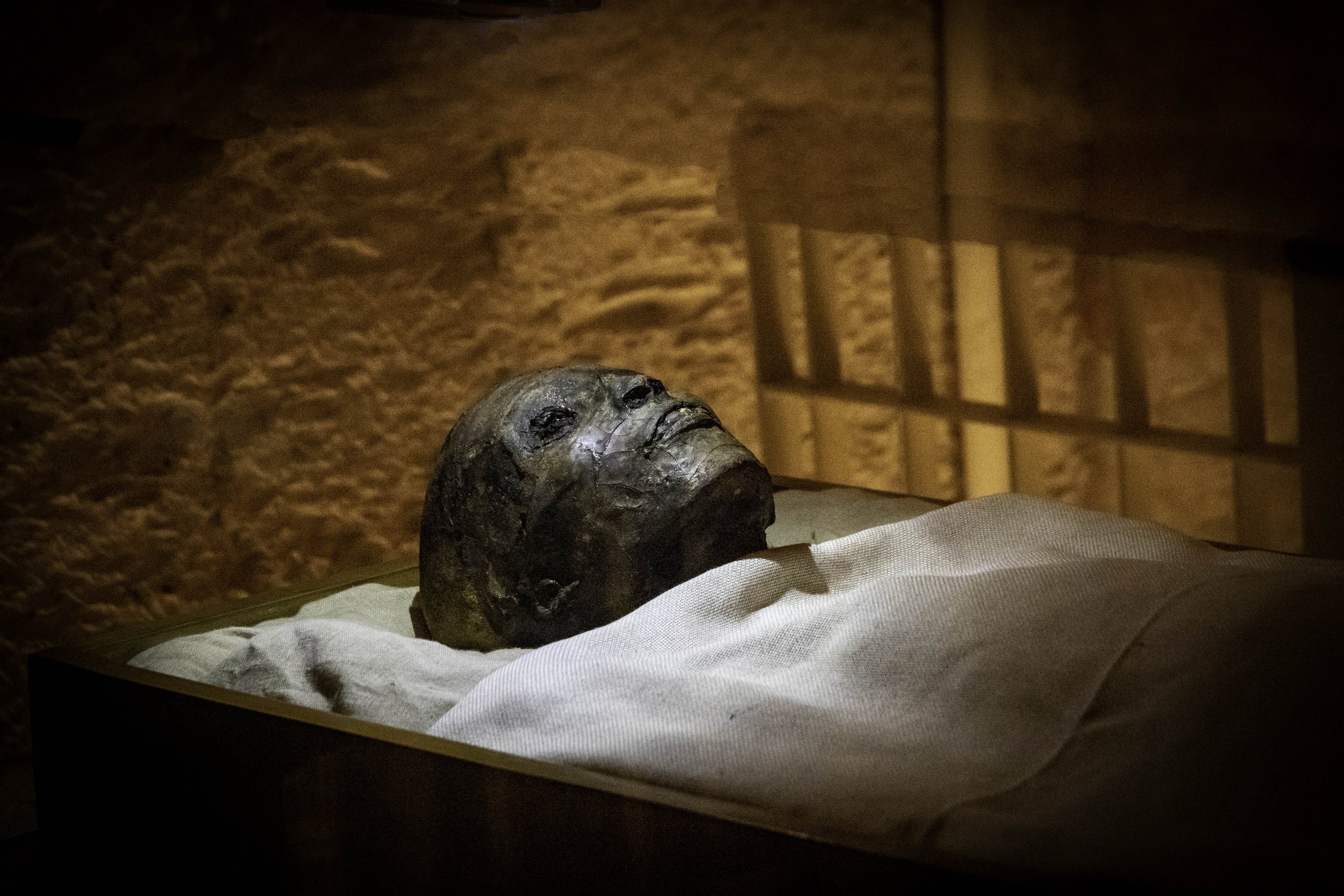The photograph features a dramatic close-up of a mummy's head, prominently positioned in the center of the image. The mummy's head, sculpted in a ghastly visage with stretched, blackened skin resembling leather, displays its glossy, almost reflective surface. Thin lips reveal portions of decayed teeth, and hollow, dark eye sockets emphasize its ancient, macabre presence. The mummy rests within a wooden sarcophagus or coffin, while a white cloth is draped over and beneath it, obscuring the body from the head down.

The sarcophagus, partially visible, extends from the bottom left and curves up behind the mummy's head, aligning with the edges of the image. The backdrop consists of a textured, stucco-like wall with a brown hue, appearing to be stone or clay, adding to the historical ambiance. Segments of the wall create shadows that intersect with the mummy’s dramatic lighting – soft illumination from above, casting subtle highlights and enhancing the eerie, solemn mood. A pole is also discernible in the upper right quadrant, descending from above and contributing an additional element to the staged setting.